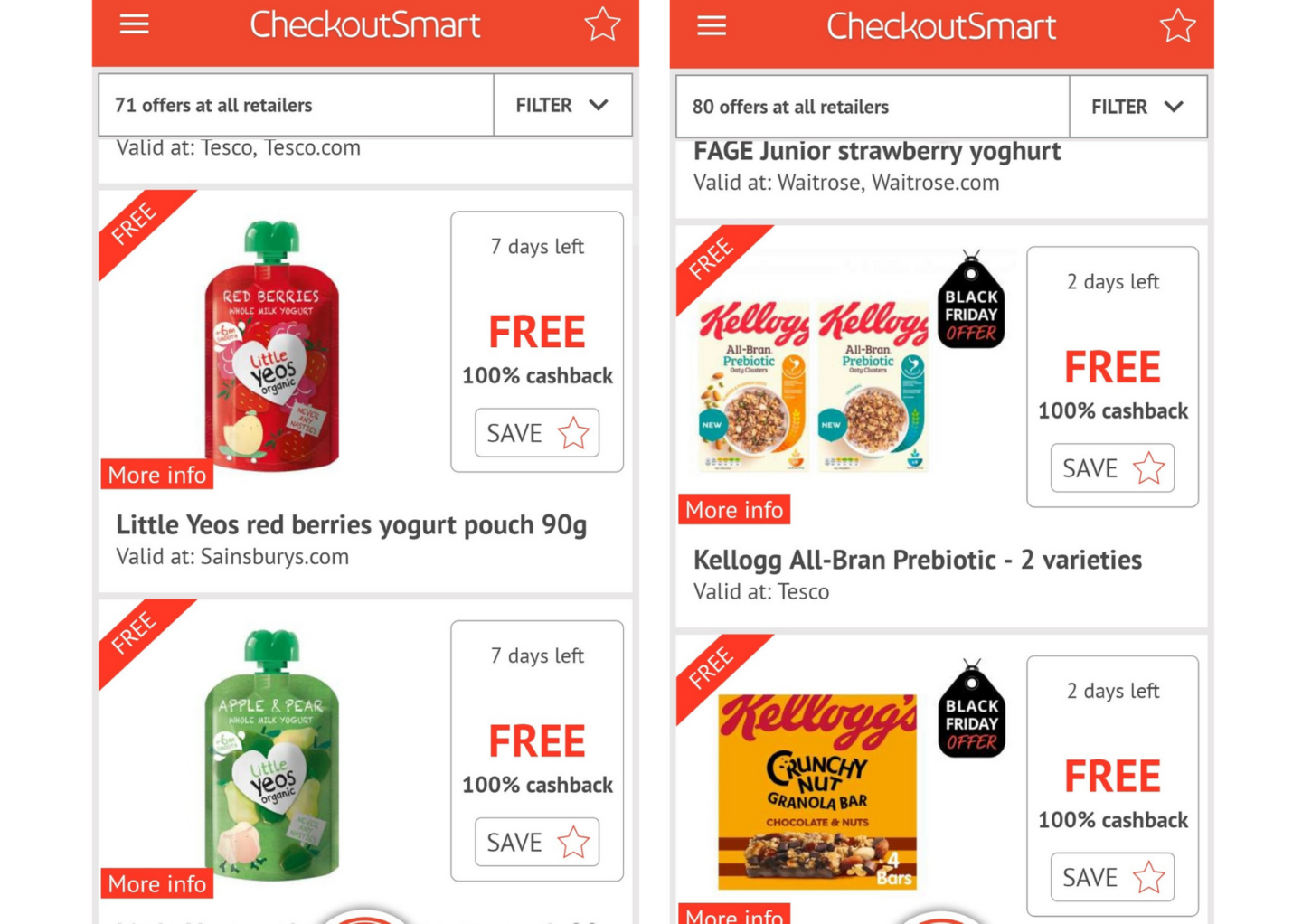This image features two side-by-side screenshots from the app Checkout Smart, which appears to be a price comparison or deal-finding platform for various retail offers. Both screenshots have identical headers displaying the app's name, "Checkout Smart," positioned at the top within a toolbar. On the left side of each header, there is a hamburger menu icon, and on the right side, there is a star icon.

In the left screenshot, the app lists "71 offers at different retailers" with an option to filter these offers. The next line notes that these offers are "valid at Tesco or Tesco.com." Below this, there are two product listings:

1. Lil' Yeo's Redberry Yogurt Pouch (90 grams): The image depicts a small red pouch with a heart design and a green cap.
2. Lil' Yeo's Apple and Peach Yogurt Pouch: Similar in design to the Redberry pouch, it features a different flavor but lacks a full description as the image cuts off at this point.

The right screenshot displays "80 offers at retailers," with an option to filter as well. Additionally, it highlights a specific offer for Fage Juni Strawberry Yogurt, valid at Waitrose and Waitrose.com. Beneath this, two more product listings are visible:

1. Kellogg's All-Bran Prebiotic in two varieties: The image shows two distinct cereal boxes featuring the well-known Kellogg's branding.
2. Kellogg's Crunchy Nut Granola Box: This yellow box showcases the familiar Kellogg's logo, indicating a granola product.

Both screenshots provide a glimpse into the array of offers and products available on the Checkout Smart app, each tailored for different retailers and displaying promotional deals on various food items.